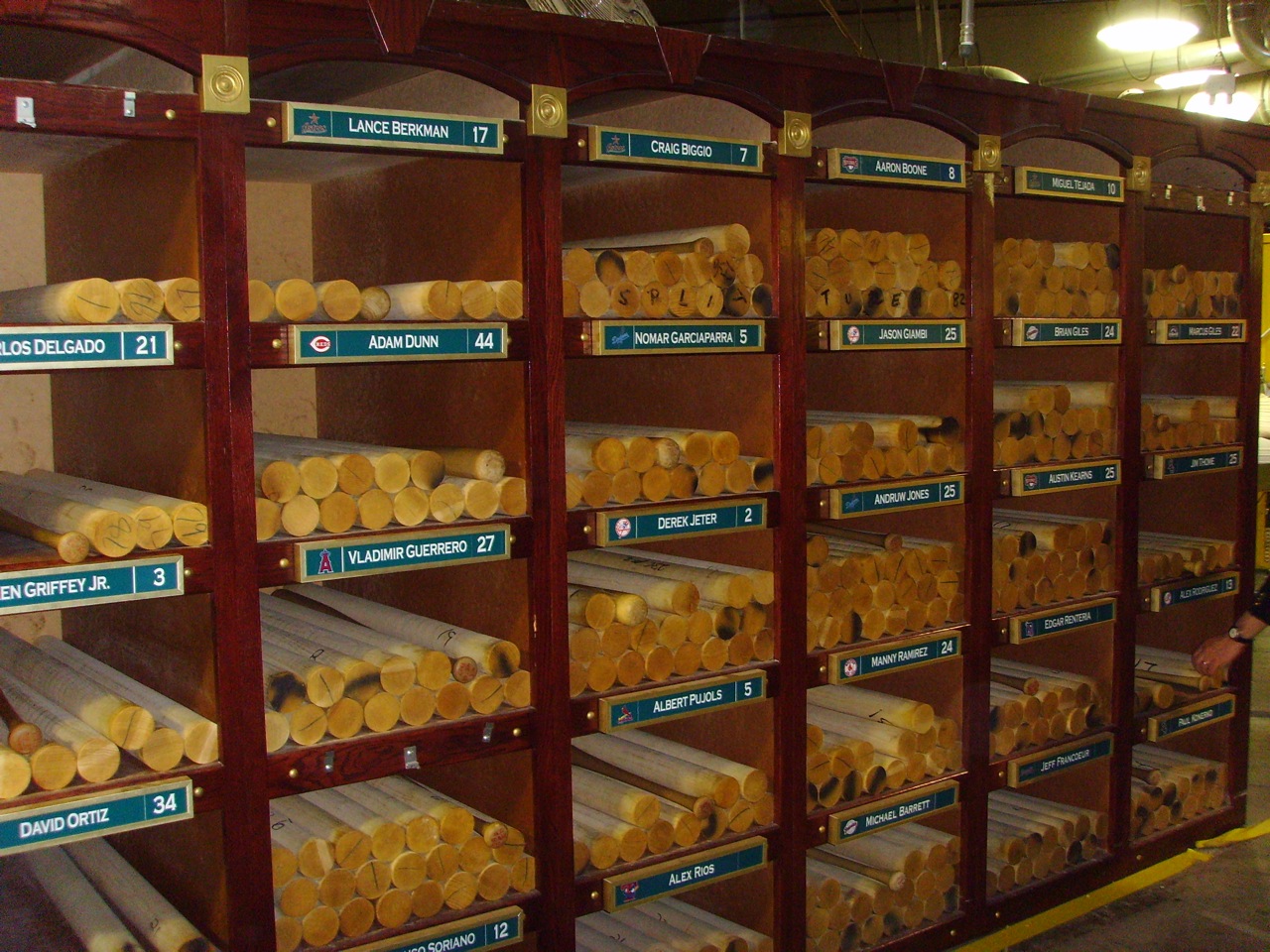In the photograph, there is a front-facing view of a shelving system crafted from dark-colored wood. The shelves are rectangular and are dedicated to storing an array of baseball bats. At the top of the image, ceiling lights faintly illuminate the scene. Each shelf is adorned with a blue nameplate featuring white text. These nameplates display the first and last names of various baseball players, their team logos to the left, and their jersey numbers to the right. Notable names like Ken Griffey Jr. (3), David Ortiz (34), Lance Berkman (17), Adam Dunn (44), Vladimir Guerrero (27), Derek Jeter (2), and Albert Pujols (5) can be identified. The rectangular compartments either hold complete bats or pieces of bats that appear to be in varying stages of manufacturing. Some of these bats may be player-used and potentially destined for auction. The overall atmosphere of the image gives a sense of deep respect for the intricacies involved in preserving and displaying the sporting equipment of renowned baseball players.